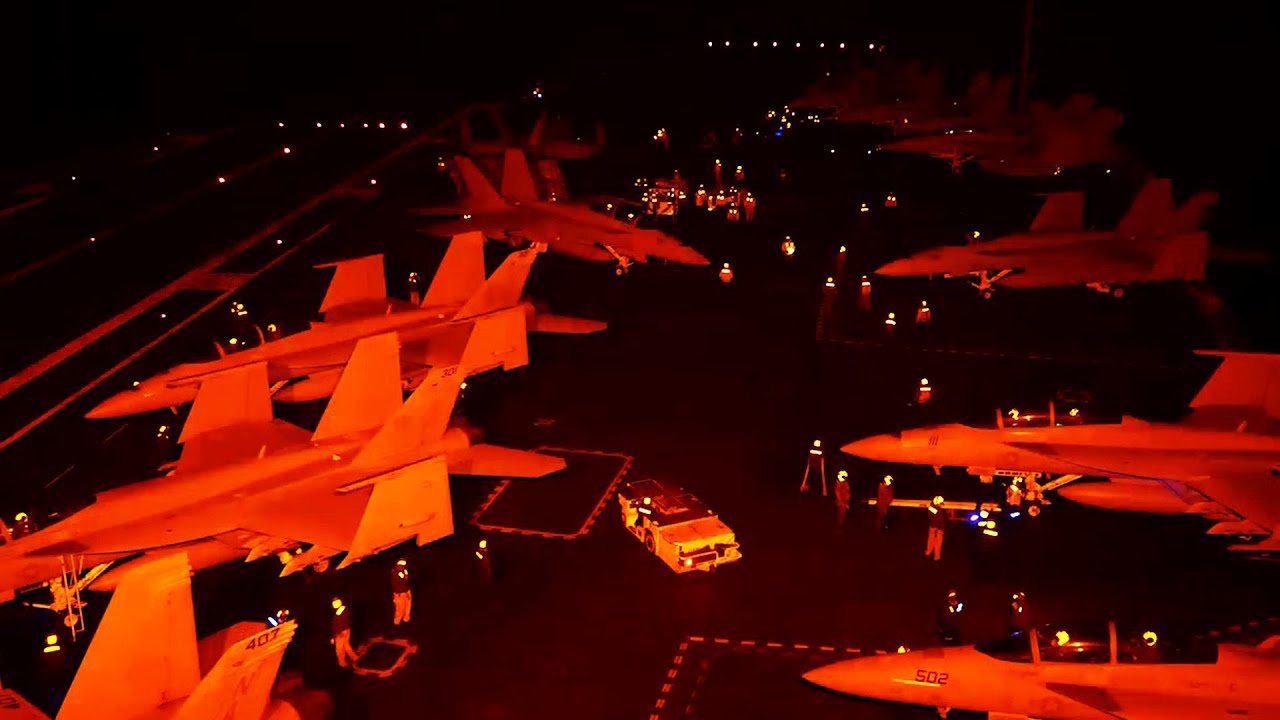This horizontal, rectangular photograph, taken at nighttime from a high vantage point—possibly an airport control tower or aircraft carrier deck—shows a dark background with solid black at the top. Small rows of lights are visible in the upper center and upper left areas, and a few scattered lights illuminate the far left side of the image. 

The primary focus is on two rows of aircraft that appear to be fighter jets. In the left row, there are five jets: the lower three are aligned and pointing to the lower left, the fourth jet faces the lower right, and the fifth jet is positioned with its back towards the camera. The right row houses seven jets, all oriented towards the left. Between the rows, in the center of the image, is a yellow vehicle, possibly a tractor used for moving aircraft, and a white car near the lower middle area with someone either entering or exiting it.

The scene is populated with dozens of people, standing around both the jets and the vehicles. They are distinguished by their glowing yellow helmets, orange or bright pants, and safety vests that are lit up in yellow. The entire area is likely covered in a smooth, possibly asphalt surface with painted lines, and ground-mounted white lights add to the nighttime ambiance.